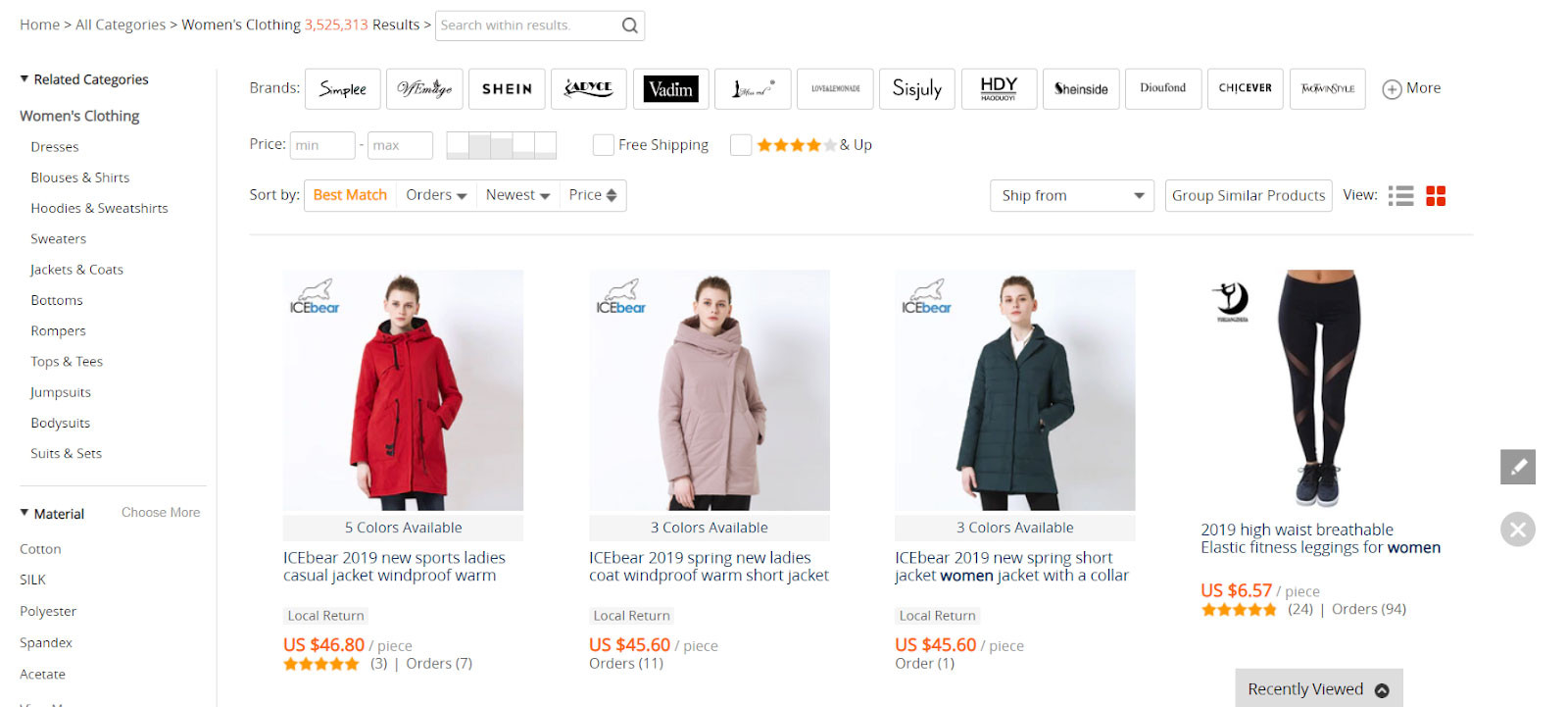This image showcases the webpage of an online clothing store, specifically highlighting selections from the women's clothing section. The page features four distinct product photographs, with the first three images displaying various women's coats while the fourth image shows a pair of women's tights.

1. **Coat 1**: The first photograph presents a vibrant red coat by the brand Ice Bear. The coat is designed with a hood and long sleeves, offering a stylish and warm option for colder weather.
2. **Coat 2**: The second image features another coat by Ice Bear, this time in a soft mauve color. This coat also includes a hood, exuding both elegance and practicality.
3. **Coat 3**: The third coat, also by Ice Bear, is a sophisticated green piece with button-up detailing. It combines classic design with contemporary flair.
4. **Leggings**: The fourth photograph showcases a pair of black women's leggings adorned with a mesh design. The brand name for these leggings is not fully legible, and they represent a blend of comfort and style.

Below each product photo, the respective prices are clearly displayed.

At the very top of the webpage, a horizontal menu lists around 12 different brands that customers can browse through. Directly beneath this menu, users have filters to refine their search by price range, shipping options (including free shipping), customer ratings, and a sorting feature with options such as 'Best Match,’ 'Orders,’ and 'Newest Price.’

On the left side of the page, an extensive menu provides further categorization within women's clothing, including specific categories such as dresses, blouses, sweaters, bottoms, tops, tees, and more, allowing for a refined and user-friendly shopping experience.